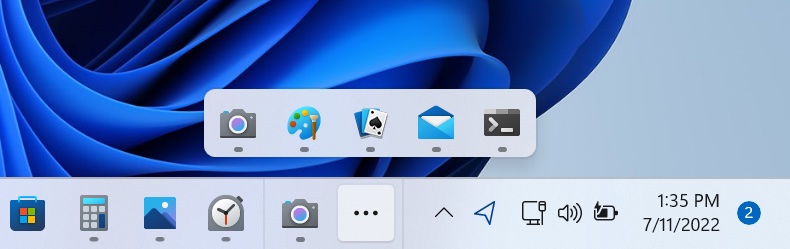This is a detailed screenshot of the bottom portion of a Windows 11 desktop screen. The top part of the image reveals a blue abstract wallpaper featuring waves that flow from the upper left to the lower right, some looping and swirling along the way. Centered at the bottom of the screen is the taskbar, a thin horizontal gray bar that spans the width of the display. 

On the left side of this taskbar, there are five icons: a Windows folder, a calculator, a desktop icon, a clock or alarm, and a camera. These are followed by a light gray square with three dark gray dots, which, when clicked, expand into a secondary gray bar above. This secondary bar contains additional icons for a camera, a painting easel, a set of playing cards, a mail icon, and a command line.

To the right of the expandable section on the main taskbar, there are five more icons, including volume control and battery status indicators. Towards the far right of the taskbar, the time "1:35 PM" and the date "7-11-2022" are displayed, and above them is a blue circle with the number "2" indicating notifications. The overall scene gives a clear snapshot of the lower-right section of a Windows 11 screen setup.